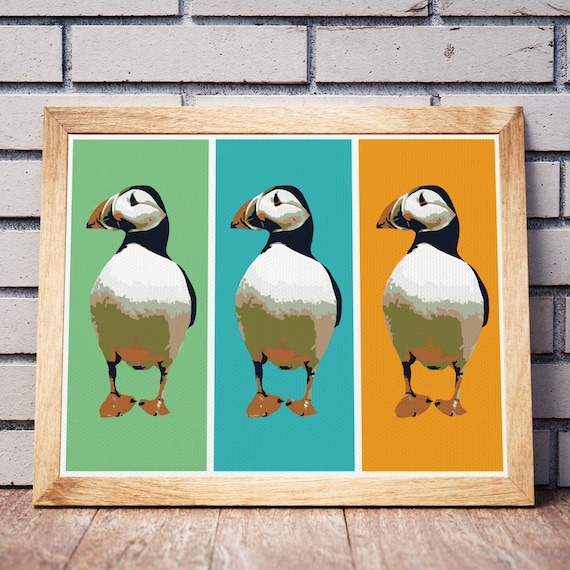The image features a framed triptych piece of art showcasing three identical puffins, each positioned within a section of the artwork divided by thin white borders. The frame is made from light wood and rests on a light brown wooden floor against a white brick wall. Each puffin, depicted with a black head, white chest and belly, black upper parts, a distinctive orange and black bill, and webbed orange feet, stands against a different colored background: green on the left, blue in the center, and orange on the right. The puffins appear to be looking off to the left, and their identical illustrations create a cohesive and repetitive visual element within the triptych format.